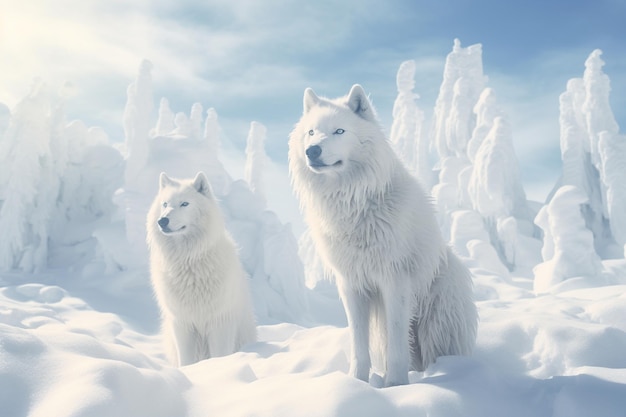In a striking and detailed artistic rendition of an arctic environment, two majestic Arctic wolves sit centrally in a snowy landscape, looking intently into the distance. The two white wolves, with their thick fur, black eyes, noses, and ears with hints of black, are positioned one slightly larger and closer than the other, with their bodies facing slightly to the viewer’s left, offering a three-quarters view of their faces and snouts. Their front paws are subtly sunken into the rocky, uneven snow beneath them. Behind the wolves stretches a breathtaking background of glaciers, ice-covered rocks, and formations resembling icy tree columns, lending a surreal and otherworldly quality to the scene. Above, the sky transitions from blue with wispy clouds to a foggy, mist-like haze, encapsulating the serene yet curious essence of the wolves as they stare out, seemingly captivated by something unknown in the distance. The combined elements of fur texture, snow details, and atmospheric conditions render this image beautifully lifelike, blurring the line between illustration and photorealism.